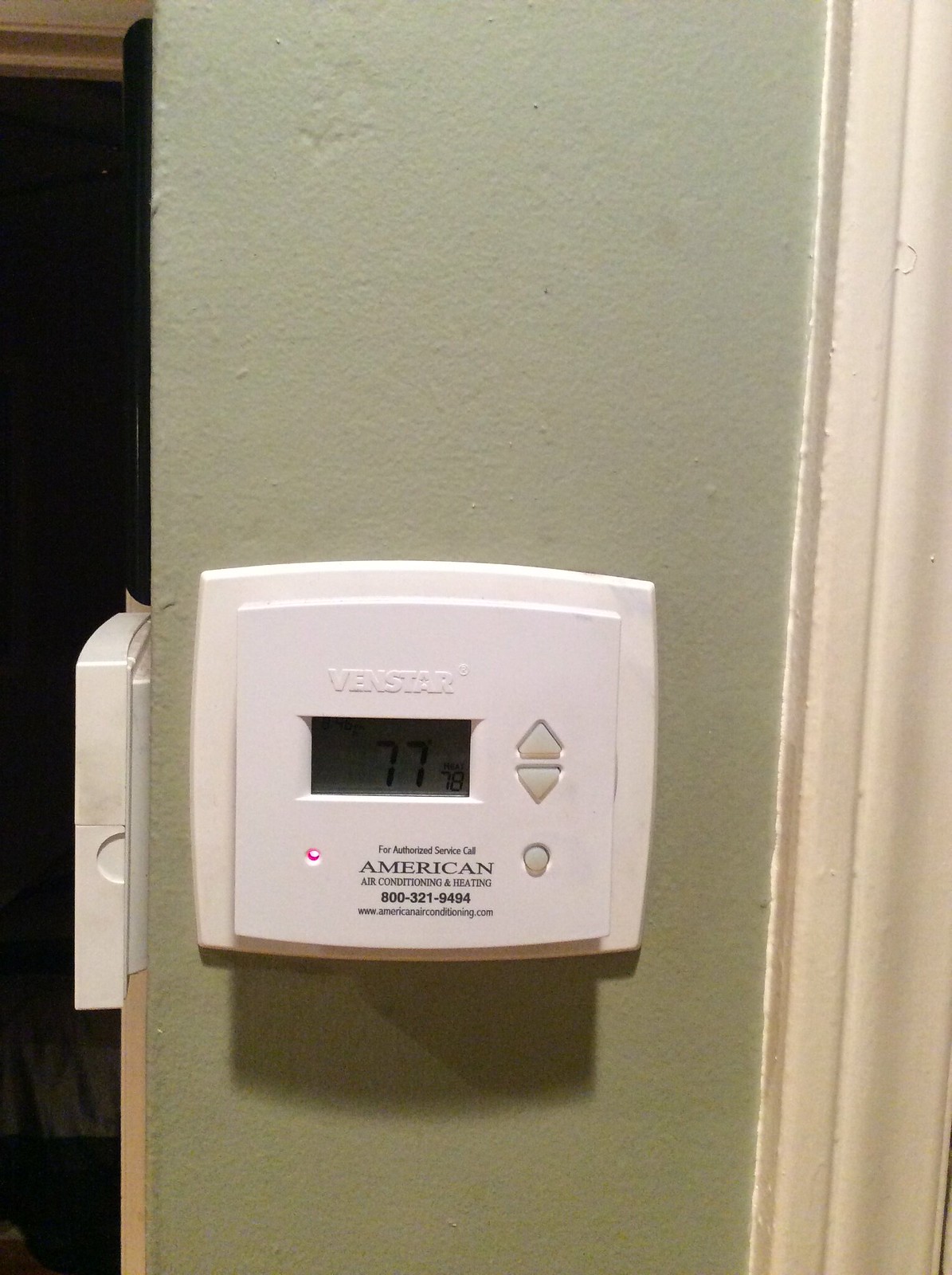This photograph features a Venstar thermostat installed on a dark avocado green pillar with tan baseboards. The thermostat's casing is an eggshell white color and includes up and down arrows along with a power button. The display shows a temperature of 77 degrees Fahrenheit. The device also bears the message: "For authorized service call American Air Conditioning and Heating, 800-321-9494, www.americanairconditioning.com." The Venstar logo is clearly marked with a trademark symbol. On the other side of the pillar, another thermostat or security pad is mounted, facing away from the camera. In the background, a room can be seen shrouded in darkness.